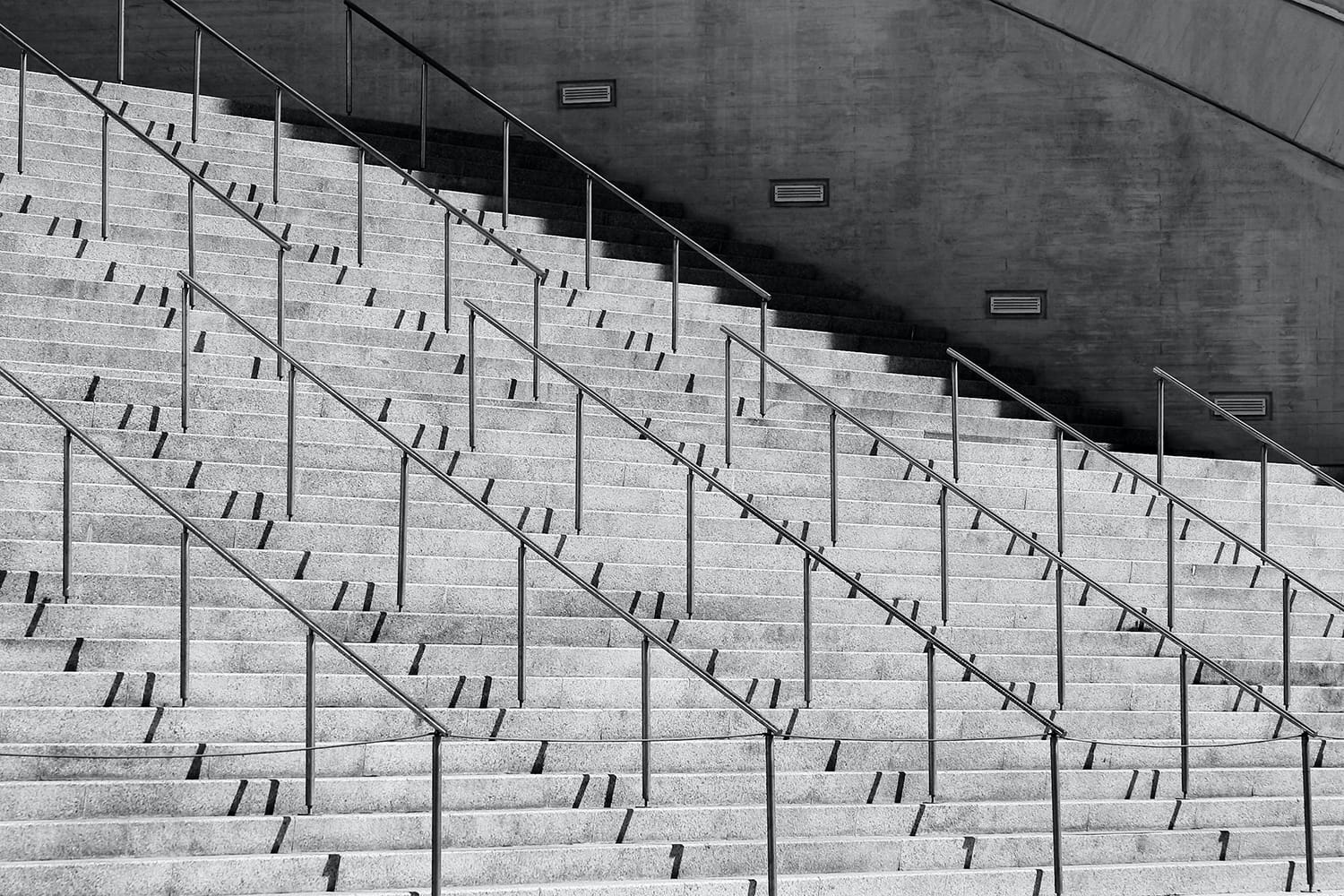This is a black and white photograph depicting a striking scene of a grand outdoor staircase composed of numerous long and wide steps, all in various shades of gray. The staircase is arranged in six distinct sets, each flanked by robust metal handrails that cast intricate shadows on the concrete surface of the steps, creating a captivating pattern. Stretching from the left to the right edge of the image, the stairs rise towards an imposing background, which is dominated by a very tall, gray brick wall. The wall is punctuated with four vents and capped by substantial stone blocks, though the top right corner is partially cut off. The steps, likely numbering around fifty, suggest an ascent to a significant structure, potentially an important building or a grand stadium. Small signs are visible along the right side of the image, adding an element of detail to the stark, industrial atmosphere of the scene.